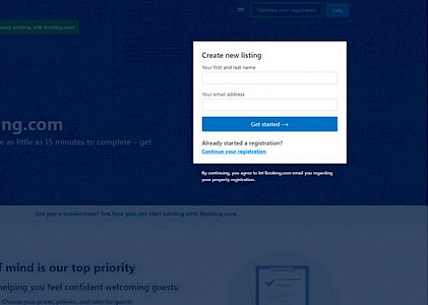This screenshot captures a website interface, specifically a registration page for listing properties on Booking.com. The focal point of the image is a white box in the center, entitled "Create New Listing," which is highlighted while the surrounding content is dimmed. The form within this box prompts the user to enter their "First and Last Name" and "Email Address," both of which have corresponding empty fields.

Beneath these fields, a prominently displayed blue button labeled "Get Started" is present. Below this button, a question reads, "Already started a registration?" followed by a hyperlink inviting users to "Continue your registration."

Additionally, there is a faded statement indicating, "By continuing, you agree to let Booking.com email you regarding your property," though the end of this statement is partially illegible. This indicates that the website's purpose is for listing apartments or hotels.

The overall background of the screen is green, while the bottom half, which is not fully visible, remains white with some obscured text. At the very top of the screen, there is a search bar, although its function or what it can search for isn't clear from the screenshot.